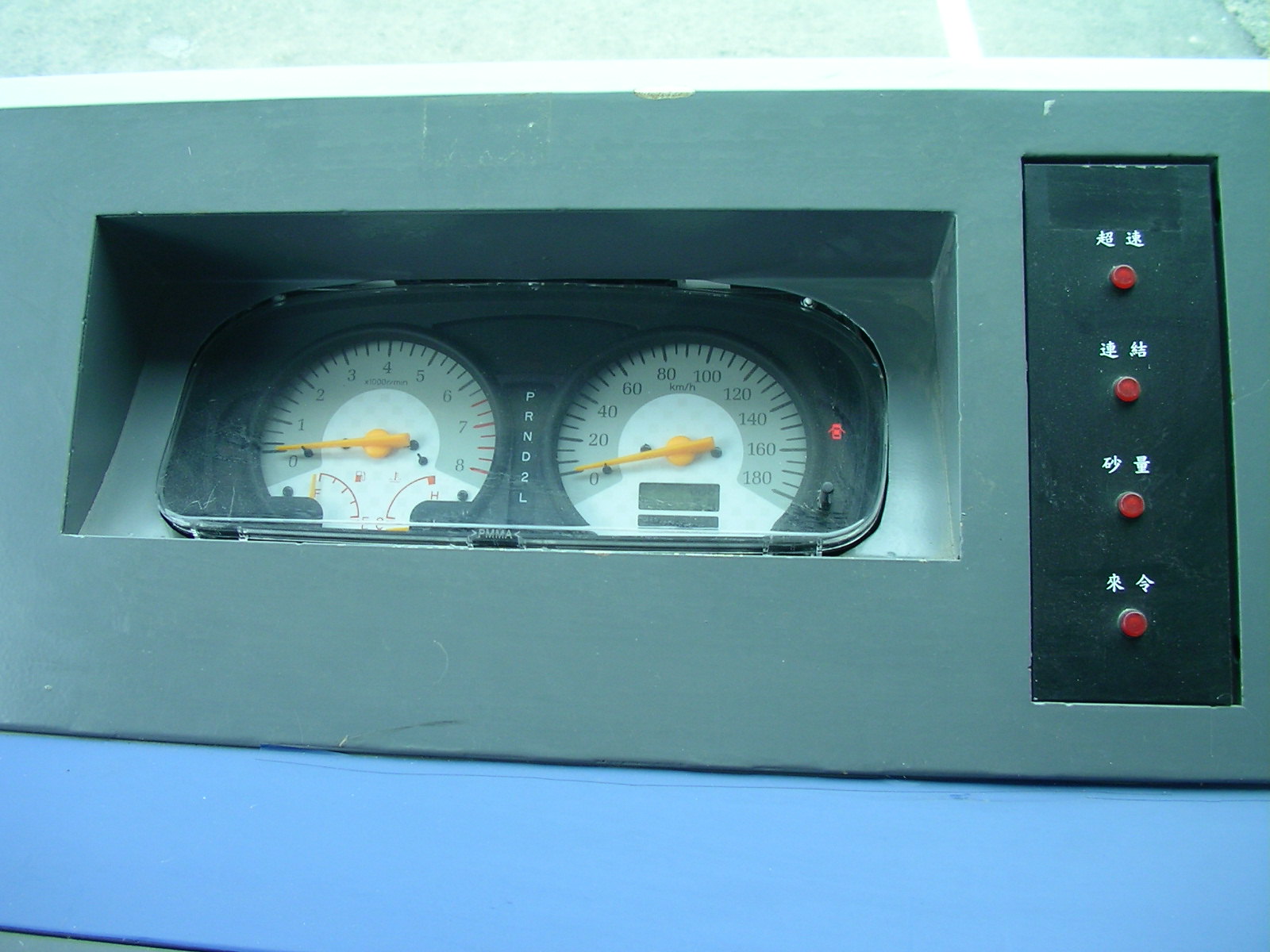The image is a slightly out-of-focus color photograph, not of the highest quality, depicting a set of dials and controls on a piece of machinery, potentially construction or automotive equipment. Encased in a gray box with a blue base, the equipment's purpose seems uncertain, possibly serving as a remote control unit. A prominent feature is a vertical black rectangle containing four red, illuminated buttons, each labeled with two Chinese characters.

To the left, there's a horizontal rectangular indentation housing two dials. Centrally located, the gear shift indicators include P, R, N, D, 2, and L, signifying park, reverse, neutral, drive, second gear, and low gear, respectively. The left dial showcases a gauge for fuel levels, marked 'Full' and 'Empty,' and another red gauge, which could indicate engine temperature. Additionally, a gauge denoted from 0 to 8, possibly a tachometer, is adjacent. 

The right dial ranges from 0 to 180, likely measuring speed in kilometers per hour, with increments of 20 (i.e., 0, 20, 40, 60, 80, etc.). Below this dial are two bars, presumably for the odometer and trip meter, accompanied by a reset button for the trip meter.

Although these instruments resemble a dashboard setup, they are not installed in a vehicle's dashboard, suggesting a testing phase or a factory setting.